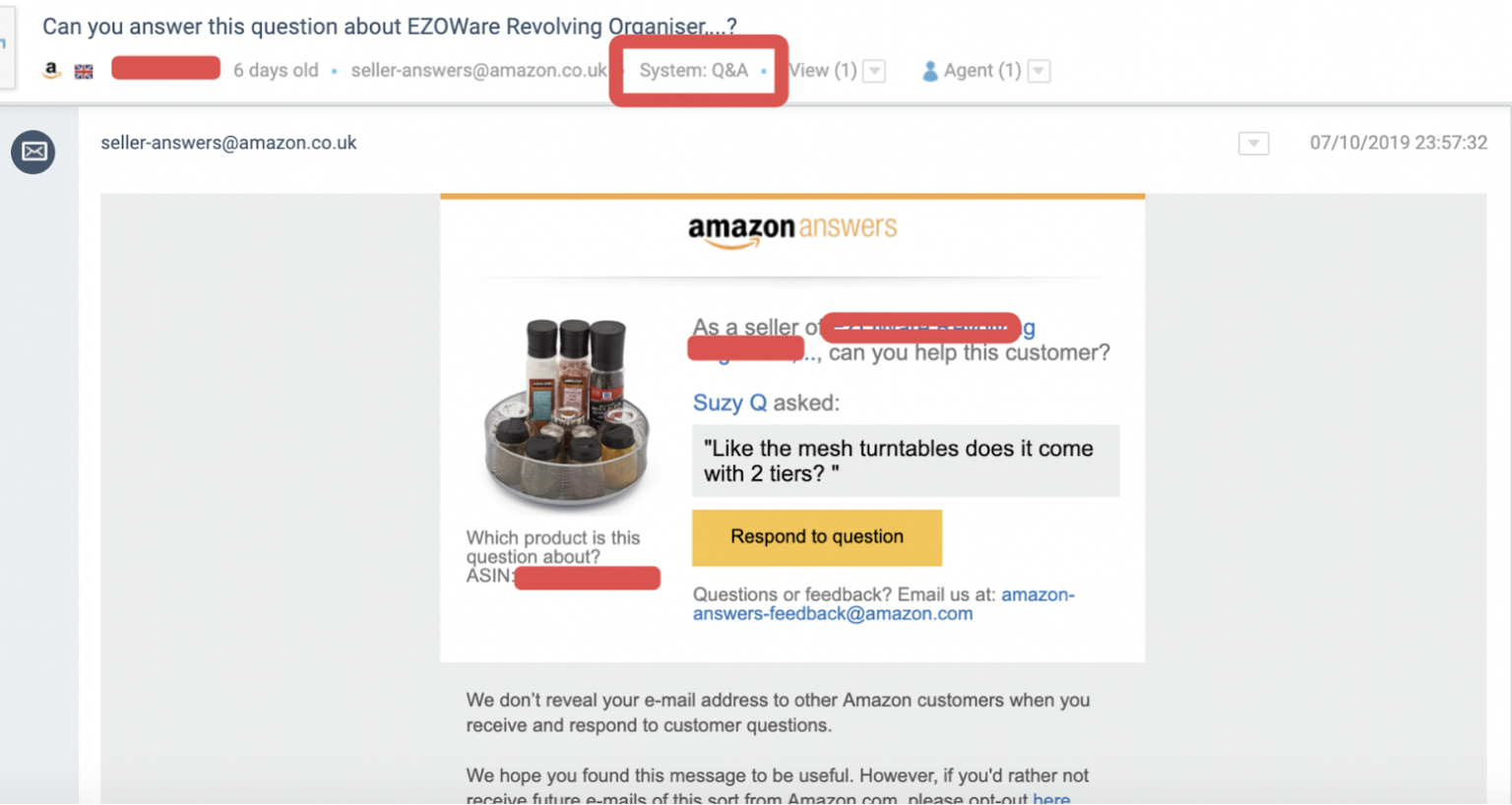Here is a detailed caption for the provided screenshot from Amazon:

---

**Amazon Screenshot Detailing a Query About a Revolving Organizer:**

The image exhibits a screenshot from Amazon's Q&A section for a product known as the EZO revolving organizer. At the top of the screenshot, a header reads, "Can you answer this question about EZO where revolving organizer?". Below this, a portion of text has been redacted with red markings. The timestamp "Six days old" is noted along with the email "seller-answers at amazon.com.uk." The section labeled "System Q&A" is highlighted with a red square.

To the left of the screen, there is a photograph featuring a circular spice organizer containing numerous bottles and jars. On the right side, text begins with "As a seller of..." but the text following is so heavily outlined that it is unreadable. Further down, additional text is crossed out in red, with the content showing, "Can you help this customer?"

The customer named Susie Q has inquired, "Like the mesh turntables, does it come with two tiers?" Below this, there is a prompt to respond to the question and contact details for feedback, listed as "amazon-answers-feedback at amazon.com."

Underneath the photograph, there is text asking, "Which product is this question about?" followed by an "ASIN" (Amazon Standard Identification Number) that has been redacted in red. Additionally, there is a disclaimer indicating that customer email addresses are not revealed to other Amazon customers and instructions for opting out of receiving future emails of this nature.

---

This caption offers a detailed description of the content and context shown in the screenshot.